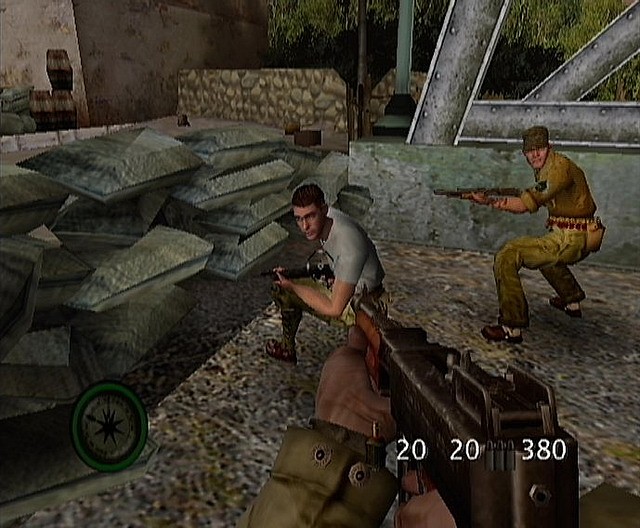A screenshot from the video game "Medal of Honor: Above and Beyond" captures a tense wartime moment viewed from a first-person perspective. The scene is set in what appears to be either World War I or II. The player, positioned as a soldier, holds a gun pointed towards several characters standing on a stone bridge. The weapon's information HUD displays an ammo count of "20/20" and a total of "380" bullets.

In the bottom left corner, a compass indicates that North is to the top-left direction of the viewer. The bridge extends horizontally, encompassing about half the image and serving as a pathway between stone-walled structures that suggest an old village or town setting. 

Two other soldiers are visible on the screen: the first is a mercenary-like figure squatting and aiming a gun towards the player, dressed in a white shirt and brown khaki pants. To his right, another soldier also squats with a gun aimed leftward. Both characters appear to be focused on the player, creating a sense of imminent conflict.

The game's graphics resemble an older generation, potentially reminiscent of PlayStation 2, noticeable by the heavy aliasing and low-resolution textures. Despite the dated visuals, the scene effectively conveys the intense and precarious atmosphere of wartime combat.